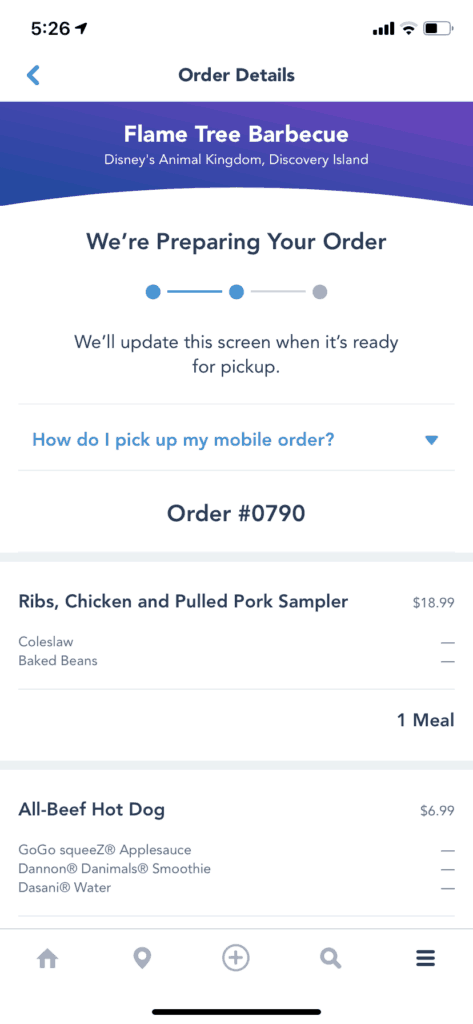In this image, we see a screenshot taken from an Apple smartphone. At the top left, the time is displayed as 5:26, while the top right features icons for the battery, Wi-Fi, and network status. The application in use shows detailed information in black text. Below this section, on a blue background with white text, it reads: "Flame Tree BBQ, Disney Animal Kingdom, Discovery Land." 

The next section features a white background with black text, stating, "We are preparing your order." There is a progress indicator with three dots, and the second dot is highlighted in blue, indicating that the order is nearing completion. Beneath this, it says, "We will update the screen when it's ready for pickup." There is a dropdown option in blue that reads, "How do I pick up my mobile order?" 

Further down, the order number "0790" is displayed in black text, followed by the ordered items: "Ribs, chicken, and pulled pork sampler $18.99, coleslaw, baked beans $1.00." Additional items include: "All beef hot dog $6.99, Gogo Squeeze S, applesauce, Danone Denimal smoothie, Dasani water." 

At the bottom of the screen, icons are visible for home, location, add, search, and the menu, with the ordering application indicated on the bottom right.